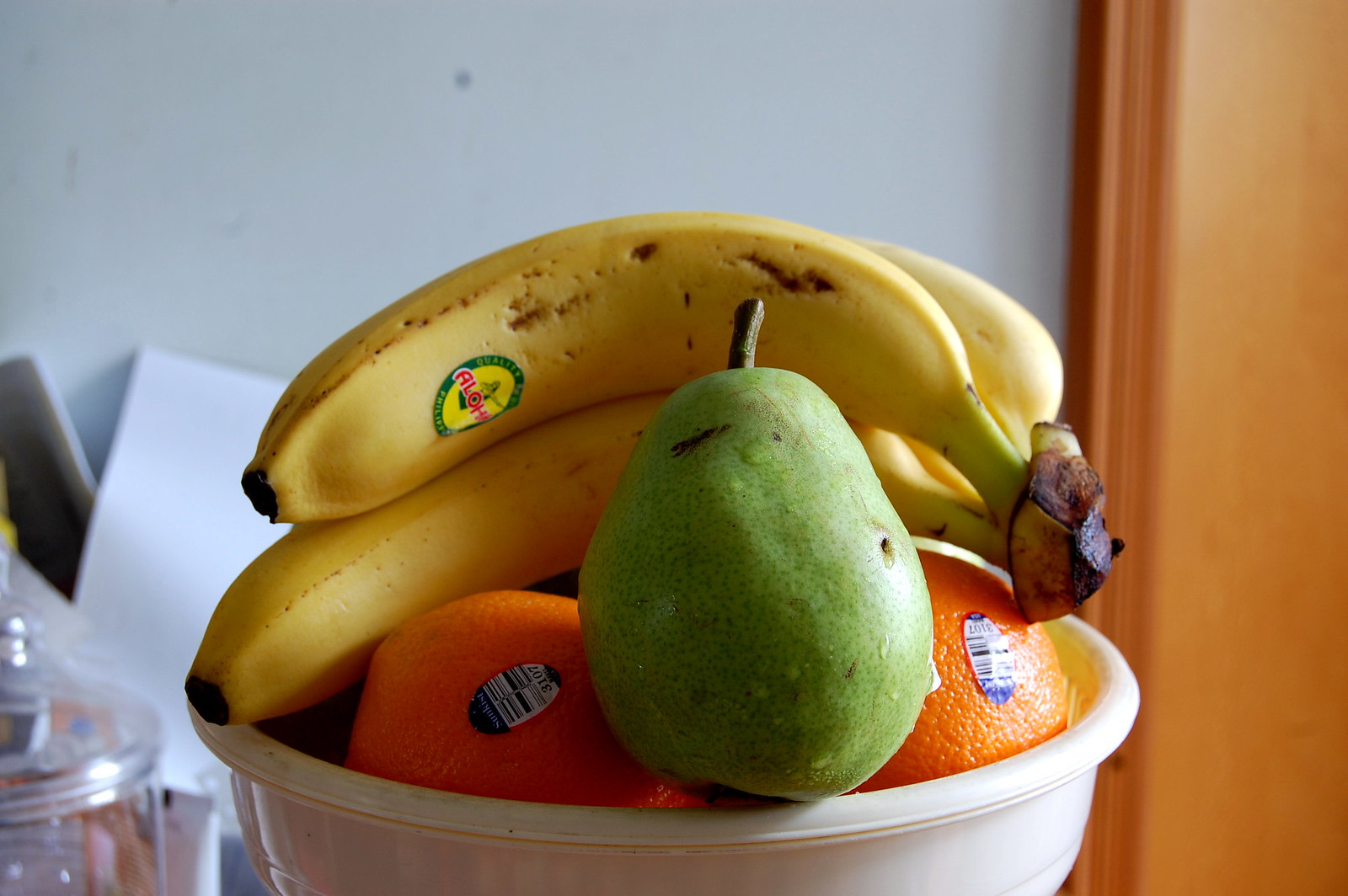The photograph features a centrally positioned white plastic fruit bowl holding a variety of fruits. At the bottom of the bowl, two oranges are visible, each adorned with a white sticker displaying a blue barcode. Resting atop the oranges is a green pear, glistening with drops of water as if freshly washed. Above the oranges and pear, a bunch of yellow bananas hangs over the side of the bowl. The top banana carries a yellow sticker with a green background that reads "Aloha" in red font. 

In the background, a plain white wall is partially obscured by out-of-focus wooden paneling on the right side. On the left side, some indistinct items appear behind the bowl, including a sheet of paper and a glass container at the bottom left. The lighting in the image is coming from the right, casting shadows on the left side of the fruit bowl, while creating a bright reflection on the right orange. This well-lit and detailed arrangement captures the freshness and variety of the fruits in a simple yet engaging setting.